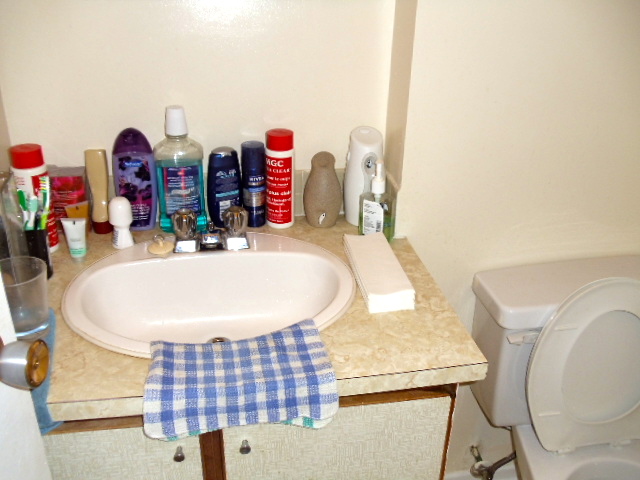In the image, a quaint, compact bathroom features a small sink set next to a diminutive toilet. The sink, devoid of counter space, is accompanied by old-fashioned faucets and a basic, dated cabinetry. A white and blue washcloth drapes over the edge, air-drying. To the right, a roll of paper towels is visible. The back of the sink is crowded with an assortment of toiletries, including a bottle of mouthwash, and two cups—one holding toothbrushes and the other likely for rinsing. The toilet, which appears to be small in size, has a beige hue and its seat is left up. The image is cropped, showing only the upper half of the toilet. The beige walls match the cabinetry, maintaining a consistent yet modest decor throughout the bathroom. A doorknob is seen on the left edge of the image, indicating the proximity of the door to the fixtures in this snug space.